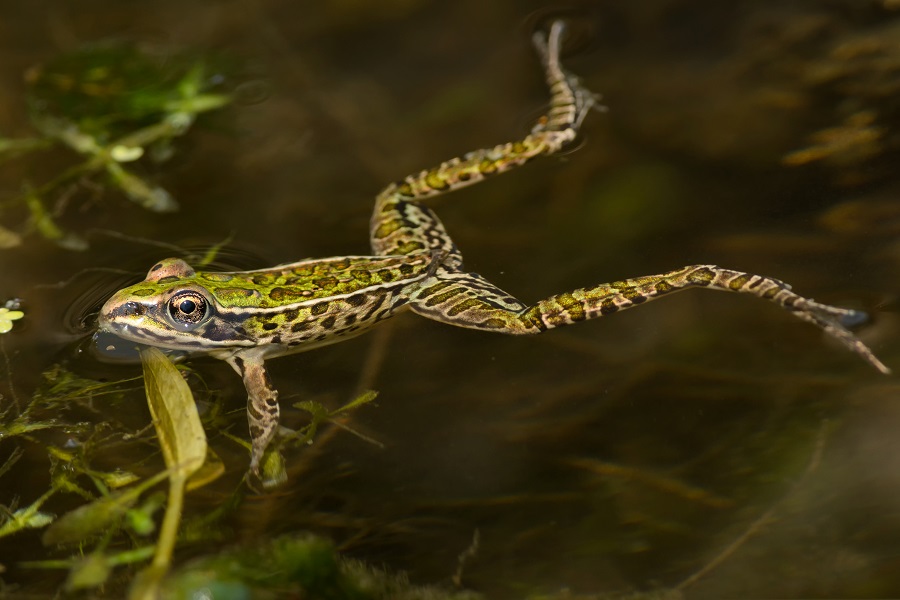In this image, we observe a small pond with water exhibiting a greenish-brown hue. Surrounding the water are various plants, displaying a mixture of vibrant green leaves and subdued brown leaves that have sunk beneath the surface. A slender, small frog is the focal point, characterized by its striking appearance. The frog's skin is a mosaic of green, black, brown, and white, with notable patches of white and gray around its face. Its large, expressive brown eyes stand out, giving it an inquisitive look. The frog's back legs are stretched out and forked, indicating a moment of relaxed repose as it seemingly enjoys its time in the water.